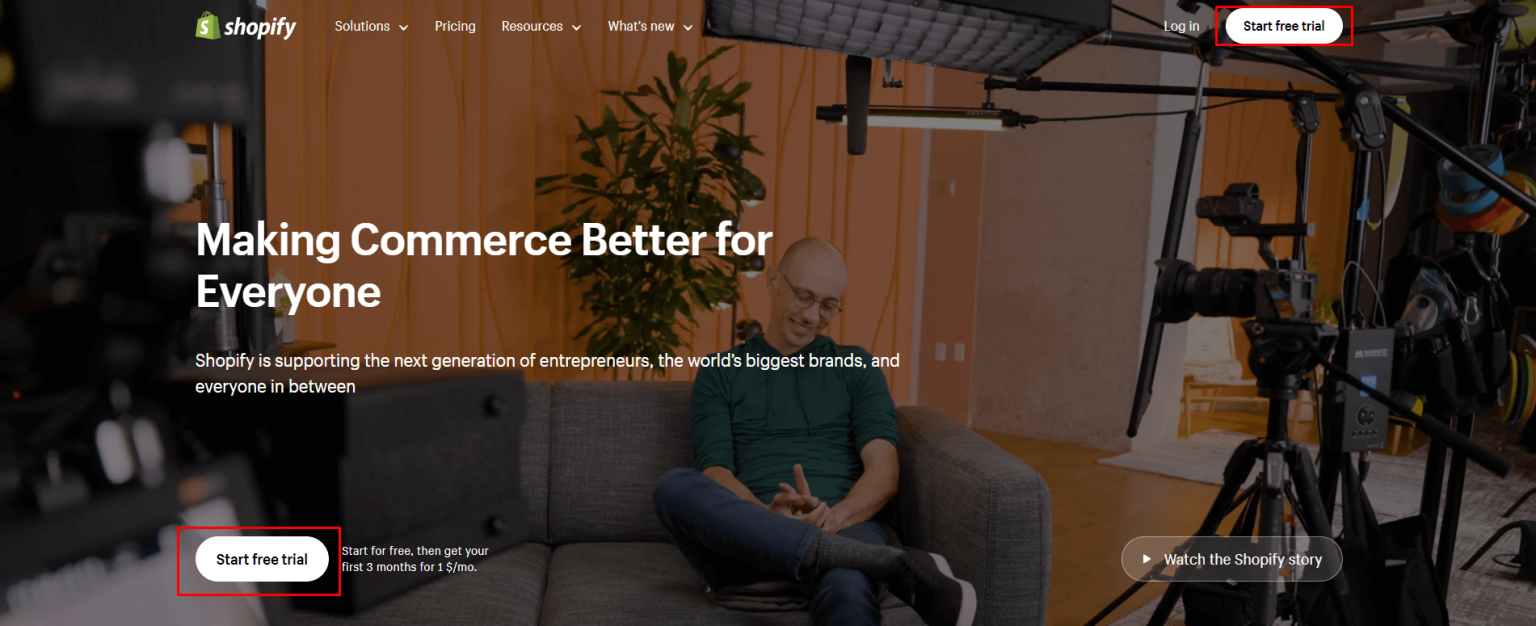This is an image of the Shopify landing page. On the left side of the header, there is a lime green shopping bag icon with an 'S' on it. To the right of the Shopify logo, the header displays four drop-down options: "Solutions," "Pricing," "Resources," and "What's New."

The main background image features a bald, lean man wearing a tight-fitting green hoodie and jeans. He is seated on a gray couch and surrounded by camera equipment and lighting. The man, who is also wearing glasses, is looking down at his fingers and appears to be smiling.

Overlaid on this background image is a prominent text message: "Making commerce better for everyone." Beneath it, in smaller text, it reads: "Shopify is supporting the next generation of entrepreneurs, the world's biggest brands, and everyone in between." 

Toward the bottom of the page is a white "Start free trial" button outlined in red. Next to it, additional text states, "Start for free then get your first three months for a dollar a month."

At the top right corner of the page, there are "Login" and "Start free trial" buttons, with the latter also being white and outlined in red. In the bottom right corner, there's a "Watch the Shopify story" play button.